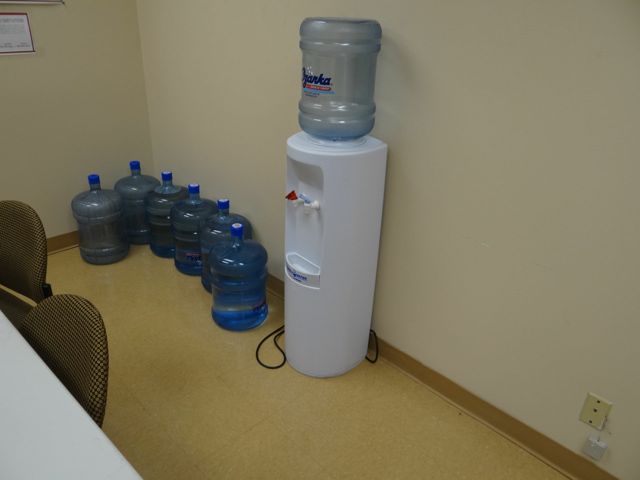This photograph, likely taken in an office space or possibly a teacher's lounge, captures a detailed view of a water station setup. The focus is on a white water cooler with a dispenser, featuring a nearly empty blue bottle inverted at the top. The cooler has three levers: one red, one blue, and one white, and a drip tray beneath to catch any spills. Adjacent to the water cooler are seven full replacement bottles, each blue with matching caps, organized neatly on the beige-peach colored floor, which has wood trim along the baseboards.

On the left side of the image, there's a white table accompanied by two brown office chairs positioned against the wall, which is painted a similar beige-peach hue to the floor. Behind the cooler, a blue cord connects to a wall outlet, alongside an old phone jack, and an additional black cord is visible. The room has an industrial feel, accentuated by details like the utility connections and the branding "Ozarka," which is printed in blue on the water bottles. The scene is well-lit, offering a comprehensive view of the room's layout and elements.